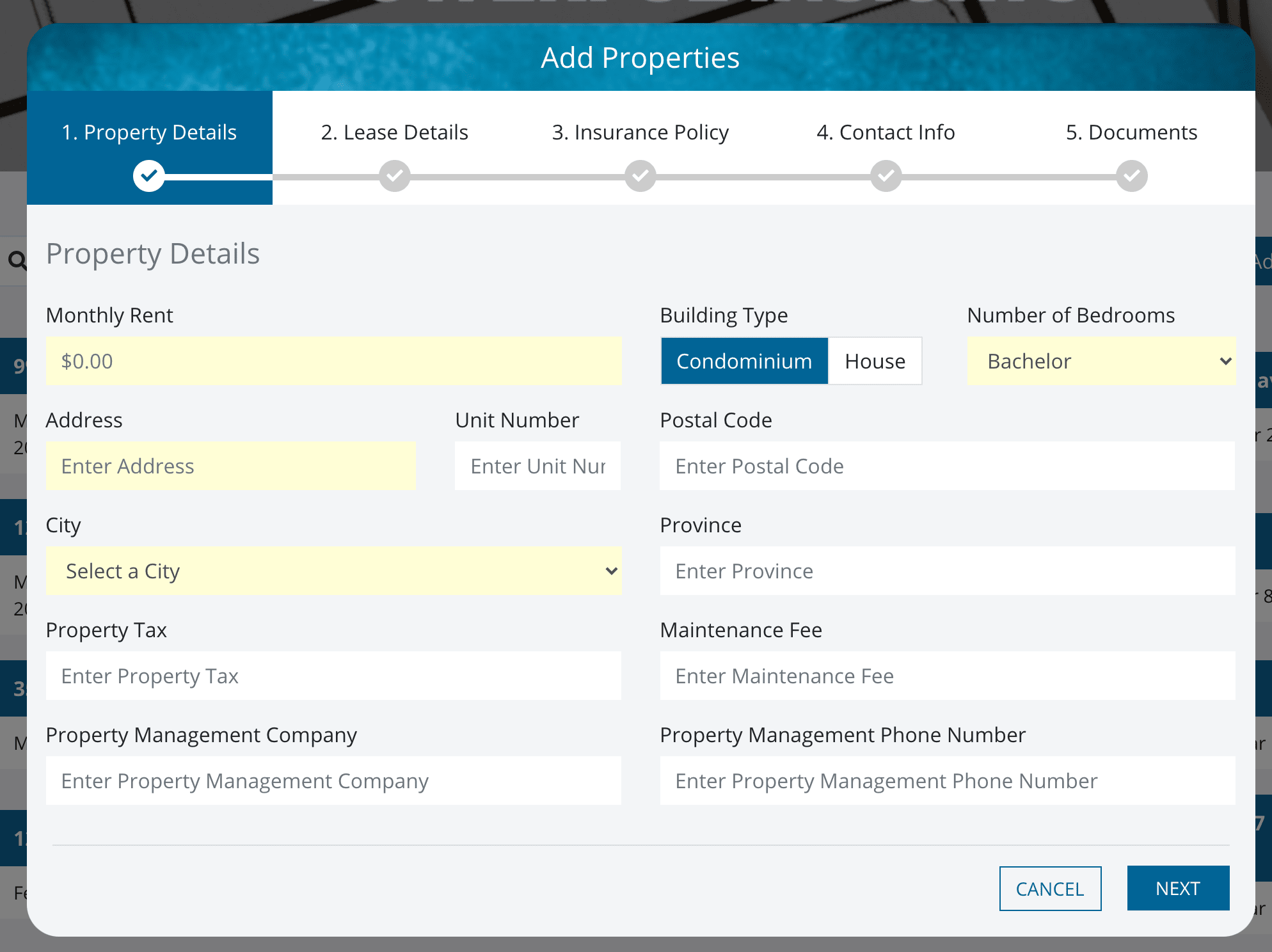The image depicts a screen capture from a webpage dedicated to managing property information. At the top of the page, there's a section titled "Add Properties" situated within a teal bluish-green speckled banner. Directly below, a progress tracker is visible, with five labeled steps connected by a continuous line: 

1. Property Details (checked and highlighted in dark blue-teal)
2. Lease Details 
3. Insurance Policy
4. Contact Info
5. Documents

Among these, only the "Property Details" section is completed and highlighted with a check mark, indicating progress.

Within the "Property Details" section, users are prompted to input various details, including the monthly rent, building type, number of bedrooms, and the address. Address fields include sections for unit number, postal code, city, and province. Further down, there are fields for property tax, maintenance fees, the property management company, and their phone number.

Two buttons at the bottom of the page, "Cancel" and "Next," offer options to either discard the changes or proceed to the next step.